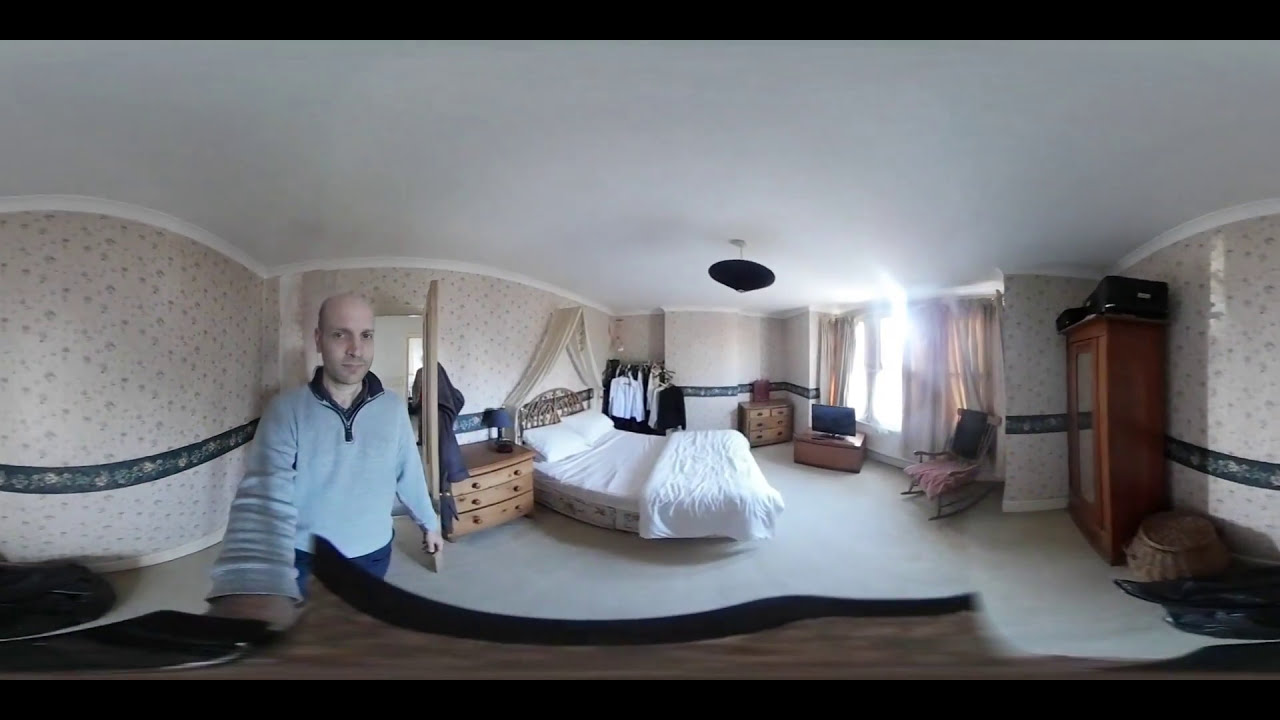This indoor panorama captures a well-furnished bedroom with a bald-headed man wearing a light blue sweater, standing at the bottom left and looking directly at the camera. The room features light-colored carpeting and semi-hardwood flooring. Dominating the center of the image is a large bed dressed in white sheets and a white comforter, turned down to reveal two pillows, and topped with an arched cloth at the headboard. Adjacent to the bed on the left side is a three-drawer wooden nightstand with a small lamp. A set of curtains and tan shades frame a bank of full-length windows, positioned near a rocking chair and a small wooden stand holding a very small TV. On the right side, there’s a larger wooden wardrobe or bureau, with a basket beside it. Clothes hang on hooks in the corner, adding to the lived-in feel. The walls are adorned with white and grayish wallpaper featuring a dark, blackish-gray border halfway down. A single black light fixture hangs from the white ceiling, illuminating the room which is decorated in hues of black, brown, light blue, dark blue, peach, and yellow. The scene is set indoors, suggesting a calm moment during the day.